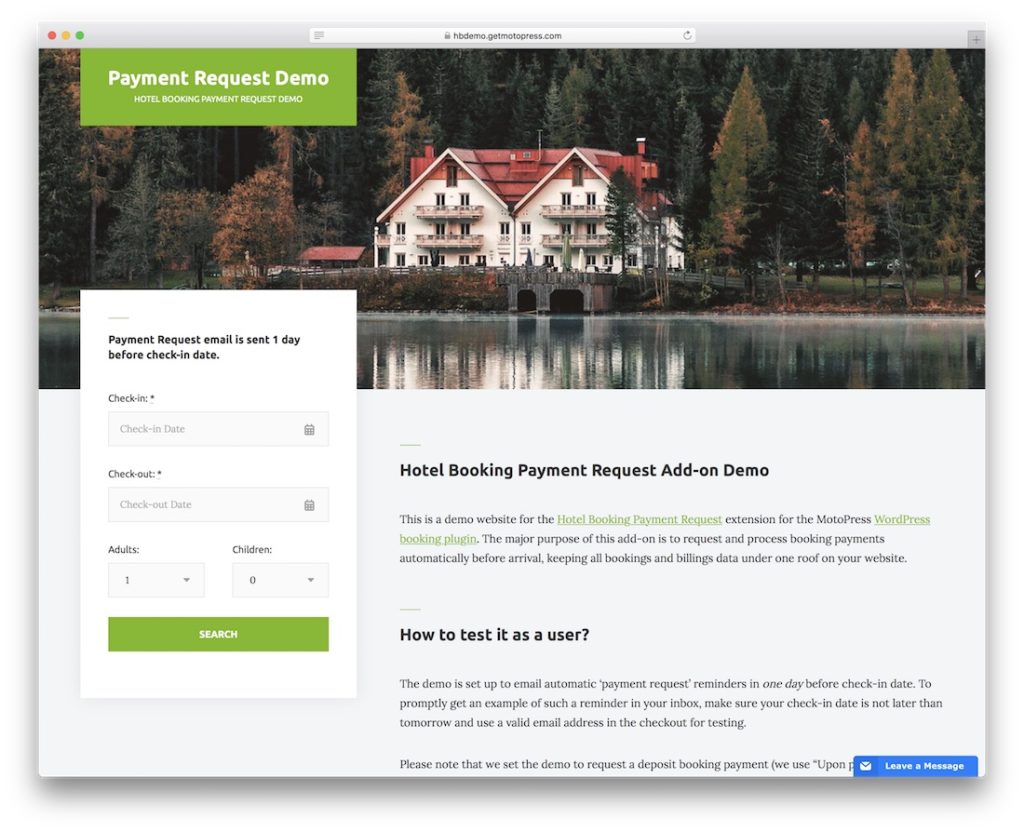**Caption:** 

In this illustrative demo for the hotel booking payment request extension from Monopress WordPress booking plug-in, various interactive elements and design features are showcased. At the top left, red, yellow, and green circles capture attention alongside the URL hbdemo.getmodelpress.com. Below, a green square labeled "Payment Request Demo" alongside text refers to the "Hotel Booking Payment Request Demo." The scene is set amidst a lush backdrop featuring vibrant foliage with green and yellow leaves, water bodies, and architectural highlights, including red roofs, white walls, balconies, and tunnels.

On the far left, it mentions a detailed procedure for the payment request email system: "Payment request email is sent one day before check-in day." Further details concerning the booking process such as "Check-in Calendar," "Checkout," "Adults: 1," "Children: 0," and a green "Search" button are captured. The demo illustrates the functionality of this add-on, emphasizing its primary goal – to automate and manage the request and posting of booking payments before guests arrive. Users can also explore features to print out bookings and billings, portraying them as being routed to an "underground roof" on the website.

For users to test this feature, the demo is configured to send automatic payment request reminders via email one day before check-in. To fully experience this, users should ensure their check-in day is imminent and verify it via their inbox. This comprehensive setup aims to efficiently streamline hotel booking payment requests.